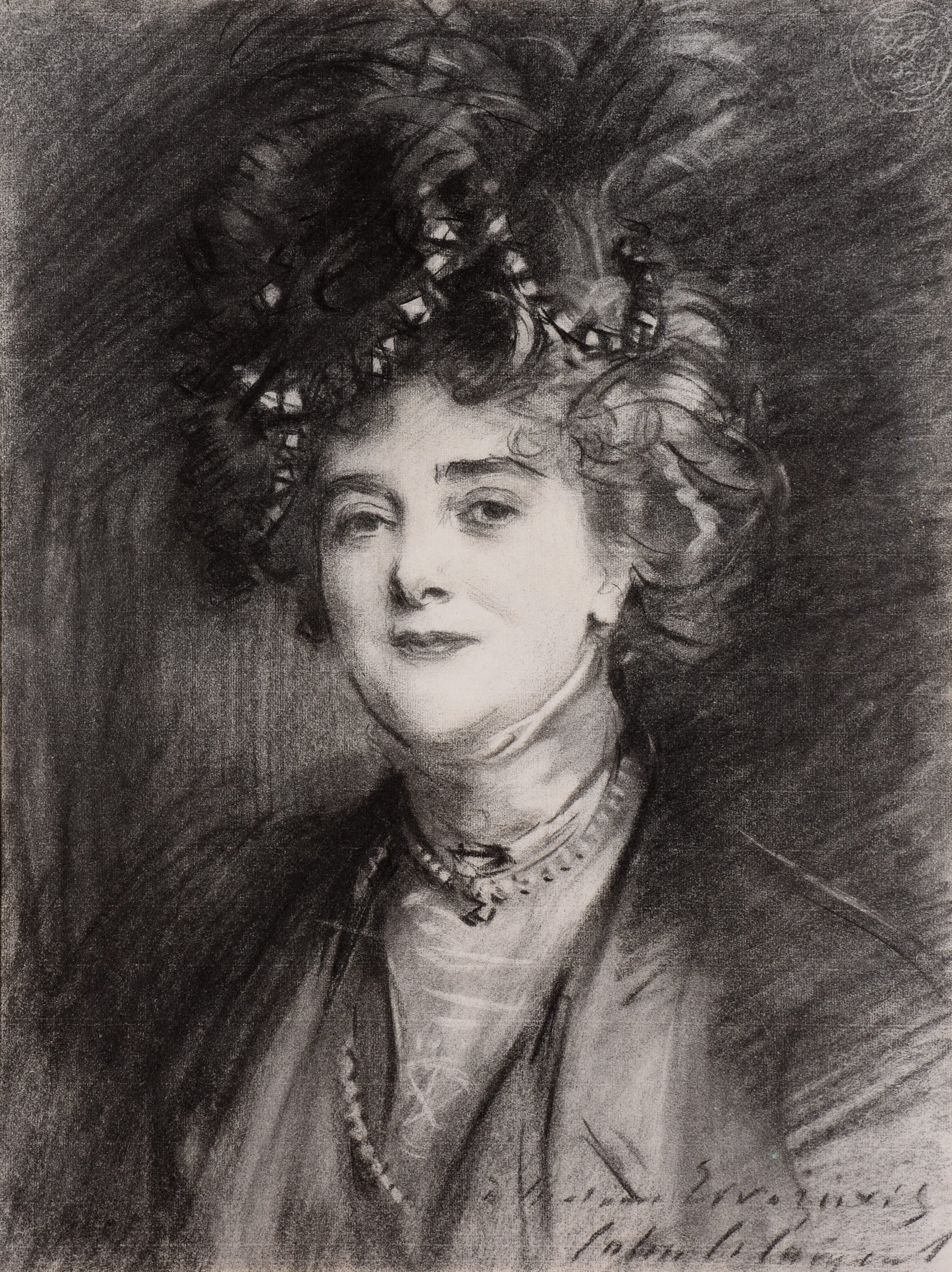This is a highly detailed pencil sketch of a woman with a striking contrast between her very fair, white face and her dark black eyes. The woman has heavy eyebrows and dark lips, giving her a bit of a smug look as she faces the viewer. Her hair is very curly, rising straight up and curling towards the top, covering the tops of her ears. She wears an elaborate hat adorned with flowers and plumes, adding to her distinguished appearance. 

Her attire consists of a high-necked blouse or dress, over which she wears a dark-colored jacket-like garment. Around her neck lies a pearl necklace, with one strand close to the neckline and another visible lower down her chest, toward the right side. Notably, there is a white circle with an X scratched into it on her chest.

The background of the sketch is composed of streaks of black and gray, resembling brushed black ink with a paintbrush, creating a stark contrast with the woman's pale face. In the bottom right corner, there is a signature comprising two lines, though it is too messy to decipher. This black-and-white image vividly contrasts shades of white, gray, and black, with the woman's face being the brightest element and some of the flowers in her hat being the darkest.